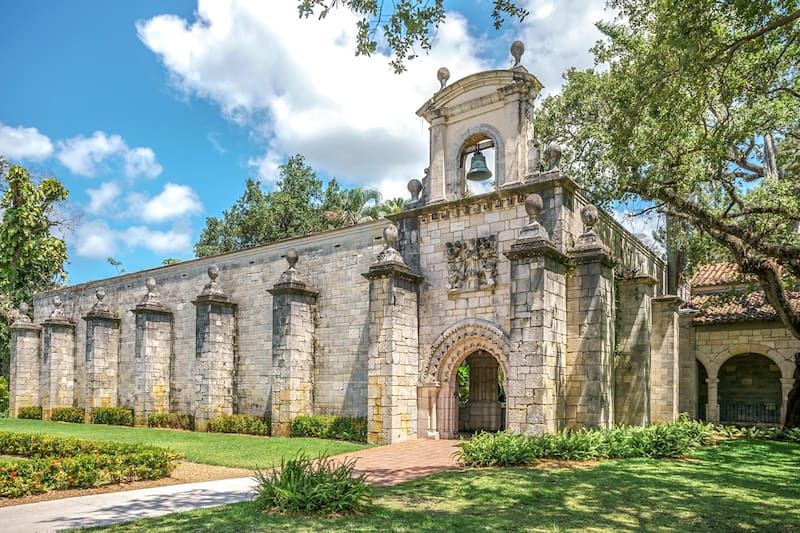This daytime photograph captures an old, weathered graystone structure, likely a Spanish mission or perhaps a church, characterized by its distinctive architectural elements. The central feature is a bell hanging from a rod perched above an arched doorway. The building's stone appears to have once been white but has aged and now bears marks of weathering, water stains, and patches of moss, lending it a grayish hue. The structure is adorned with numerous pillars, each topped with a round ball, contributing to its historic and stately appearance. Surrounding the building are lush green trees and neatly maintained garden beds. The scene is set against a blue sky dotted with white, puffy clouds. A well-defined pathway leads up to the entrance, enhancing the inviting yet serene ambiance of the setting.